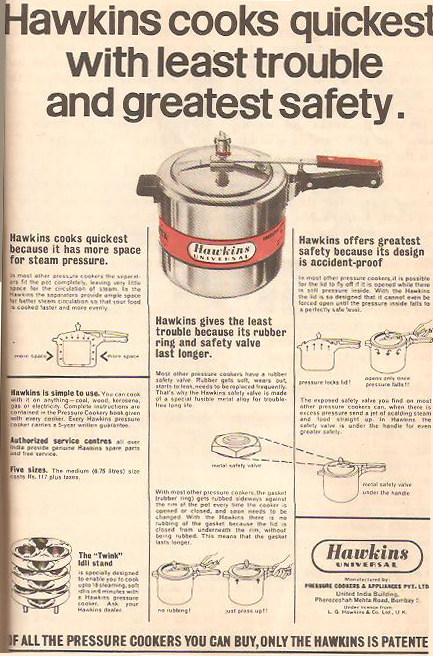The promotional image is a vertically rectangular print piece with a light peach to pinkish flesh-tone background. A thin border frames the image on the left and bottom edges. Positioned just above center is a metallic silver pressure cooker, featuring a black handle and a red band around its midsection that reads "Hawkins Universal" in black text. The cooker also has a reddish handle for lifting the lid.

At the very top of the image in black text, a bold slogan announces, "Hawkins cooks quickest with least trouble and greatest safety." Surrounding the cooker are various bits of text promoting its features: on the left, it states, "Hawkins cooks quickly because it has more space for steam pressure." Below the cooker, it explains, "Hawkins gives the least trouble because its rubber ring and safety valve last longer." To the right, it asserts, "Hawkins offers greatest safety because its design is accident-proof."

Additionally, the image presents various smaller illustrations and details about the Hawkins pressure cooker’s design and functionality, such as its simplicity of use and the presence of authorized service centers. At the bottom, the concluding message reads, "Of all the pressure cookers you can buy, only the Hawkins is patented," emphasizing the uniqueness of the product. This vintage promotional piece effectively highlights the superior attributes of the Hawkins Universal pressure cooker.